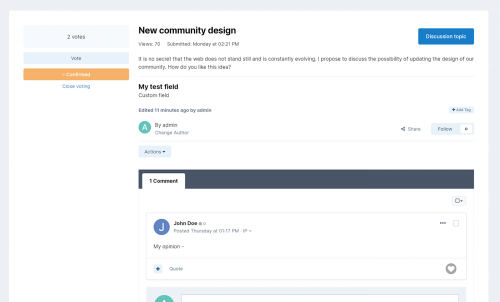The image is a screenshot taken from a website viewed on a computer. At the top center of the screen, "New Community Design" is prominently displayed in black print. On the left side, there is a section indicating "2 votes," accompanied by options to "Vote" and "Start Voting." Above this section, there is an orange clickable box. 

The middle section of the screen contains a text box with the following message: "It is no secret that the video does not stand still and is constantly evolving. I propose to discuss the possibility of updating the origin of our community. How do you like that idea?"

At the bottom of the screen, users are given the opportunity to share their opinions. There is one visible comment made by a user named John Doe, represented by a blue circle with a white "J" inside. The comment starts with "My opinion" but is truncated, preventing the full opinion from being read.